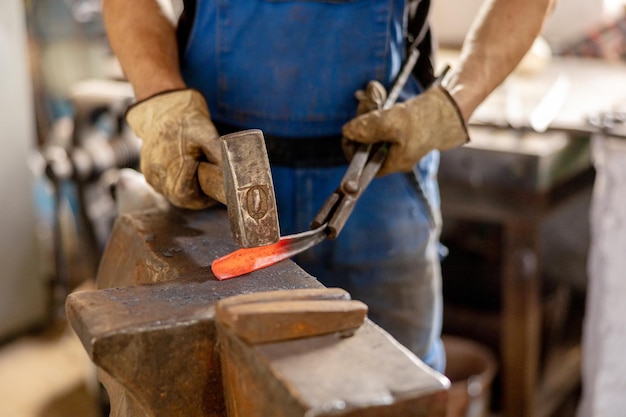In this detailed photograph, an industrial workshop serves as the backdrop where a man is intensely focused on a metalworking task. Clad in blue jean overalls and a blue t-shirt, paired with a blue and black apron, the man is equipped for a labor-intensive job. His dirty, sweaty white working gloves signify the rugged nature of his work. The image captures him from the waist down, emphasizing his strong, tanned arms and light-colored skin. 

On an iron table in front of him lies a piece of red-hot metal held steady by pliers in his left hand. With his right hand, he wields a hammer, poised to shape the heated metal through repeated blows. The metal's glowing, molten tip highlights the intense heat involved in this process. The background, though blurred, reveals an assortment of workshop tables, machinery, buckets, and tools, further cementing the setting as a busy, well-used industrial environment. This vivid scene captures the meticulous skill and dedication involved in the art of metalworking.